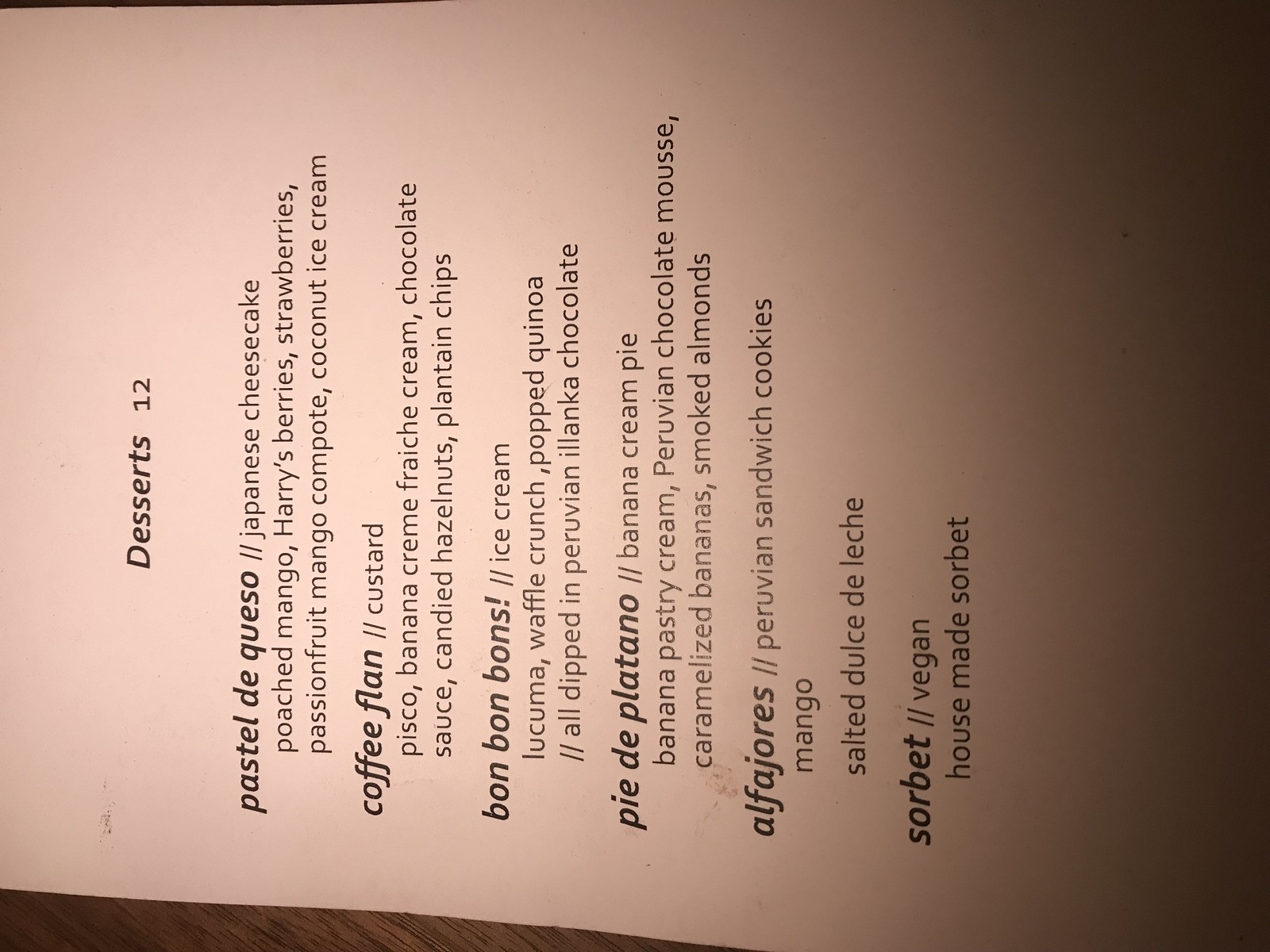A horizontally oriented photograph captures a restaurant menu laid out flat on a wooden surface, though the dim lighting makes it somewhat challenging to read. Tilting the head to the left reveals a section titled "Desserts," with a price of $12 for each item listed below. The first offering, "Pastel de Queso," described as Japanese cheesecake, is accompanied by poached mango, Harry's Berries strawberries, passion fruit, mango compote, and coconut ice cream. Next is "Coffee Flan," which consists of custard, pisco, banana, crème fraîche, chocolate sauce, candied hazelnuts, and plantain chips. Following that, "Bonbons" are presented as ice cream bonbons with lucuma, waffle crunch, and popped quinoa, all dipped in Peruvian Illanka chocolate. "Pie de Plátano" is the next item, a banana cream pie featuring banana pastry cream, Peruvian chocolate mousse, caramelized bananas, and smoked almonds. Another choice, "Alfajores," are Peruvian sandwich cookies filled with mango and salted dulce de leche. Lastly, the menu offers a vegan, house-made sorbet.